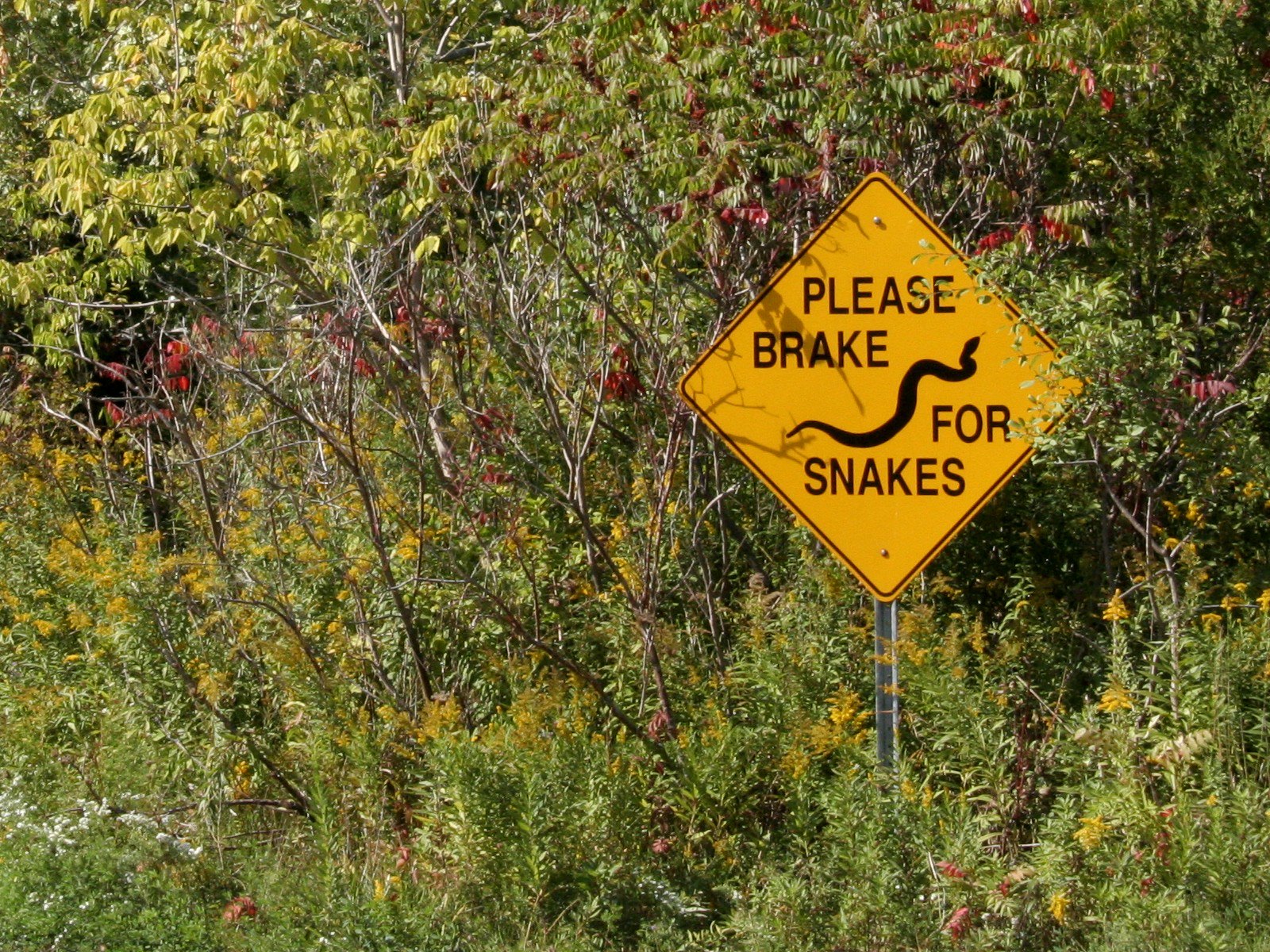In the photograph, a dense, foliage-rich background comprised of greens, golds, reds, and browns creates a vibrant and natural setting. Among the foliage, on the left-hand side of the image, stands a diamond-shaped, mustard-yellow sign mounted on a metal pole. The sign features a prominent black border around its edges and bears a distinct warning message in block letters, "PLEASE BRAKE FOR SNAKES." Below the text, on the right-hand side and near the bottom, a black snake slithers diagonally towards the upper right corner of the sign. The combination of the lush vegetation and the conspicuous sign creates a striking contrast in the scene.